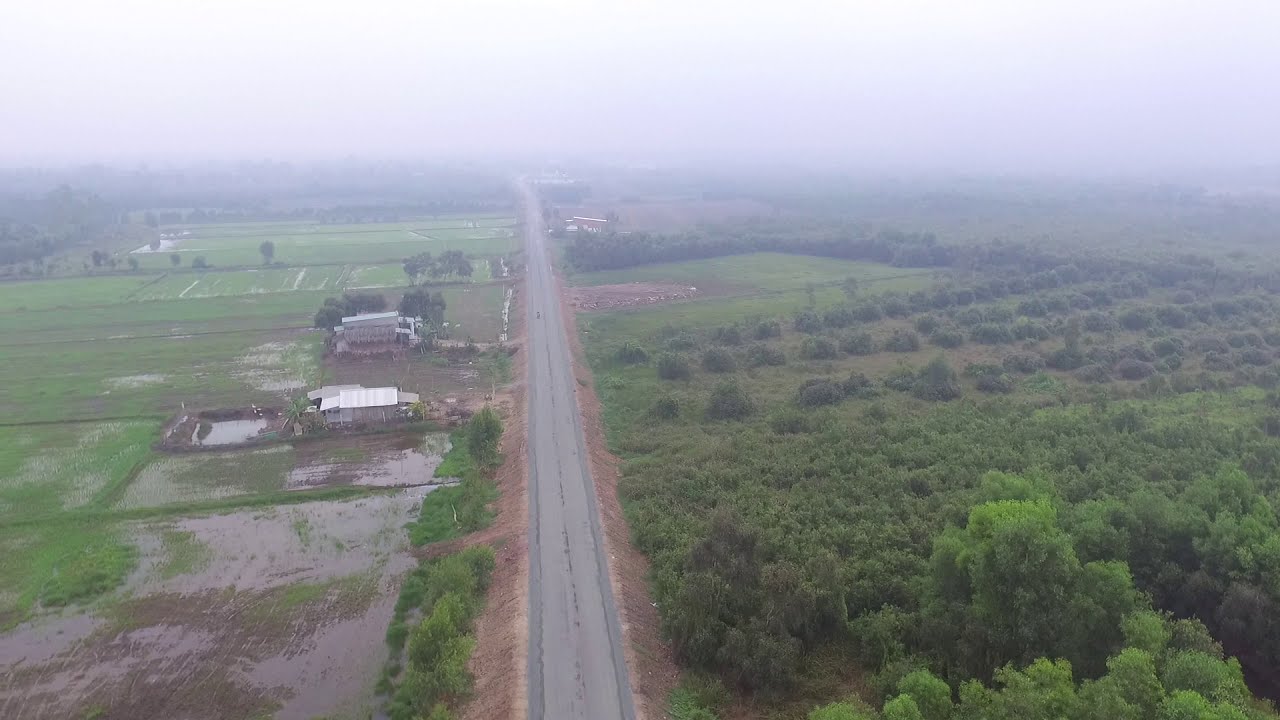The image captures a high-angle aerial view, likely taken from a drone, looking down at a country road meandering through a rural landscape. The road, which appears paved yet in poor condition without visible lines or markings, runs straight and long into the hazy, mist-filled distance. To the road’s immediate sides, dirt slopes give way to distinct scenery on either hand.

On the right, the land is typified by mostly unkempt green vegetation, including low-lying shrubs and trees which may be arranged in rows, hinting at a possible orchard or vineyard. The vegetation transitions into a more structured grassy area and clusters of trees further ahead.

Conversely, the left side features traditional farmland with patches of land segmented like a jigsaw, possibly for planting different crops. A few silver-hued barns add to the pastoral setting, and a small pond indicates potential flooding or marshland farming activity, such as rice cultivation. The ground appears saturated, suggesting recent heavy rainfall or inherent waterlogging. The expansive rural canvas is wrapped in a subdued light, owing to a foggy sky that slightly obscures the overall clarity of the scene.